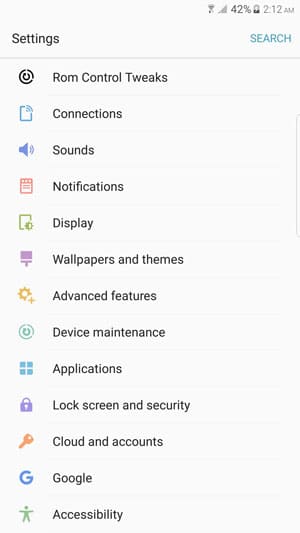Screenshot of a Mobile Phone Settings Page

The image is a screenshot of a mobile phone's settings page, displayed against a uniformly gray background. In the top right-hand corner of the screen, the battery level is shown as 42%, accompanied by a battery icon. The time displayed is 2:12 AM. Below this information, there's a blue "Search" label with the "Settings" title located on the left-hand side, separated by a grayish line. 

The settings menu is organized into various categories, each with distinct icons: 

1. **ROM Control Tweaks**
2. **Connections** 
3. **Sound**: Represented by a blue microphone icon.
4. **Notifications**: Symbolized by a pink notebook icon.
5. **Display**: Illustrated with a green document icon.
6. **Wallpapers and Themes**: Marked by a purple brush icon.
7. **Advanced Features**: Indicated by a gold gear and a plus sign icon.
8. **Device Maintenance**: Depicted with two concentric bluish circles.
9. **Applications**: Shown with four blue squares.
10. **Lock Screen and Security**: Denoted by a purple lock icon.
11. **Cloud and Accounts**: Signified by a reddish key icon.
12. **Google**: Represented by a blue capital "G."
13. **Accessibility**: Shown with a green stick figure with outstretched arms.

The organization of icons and text provides clear and intuitive navigation through the various settings of the device.